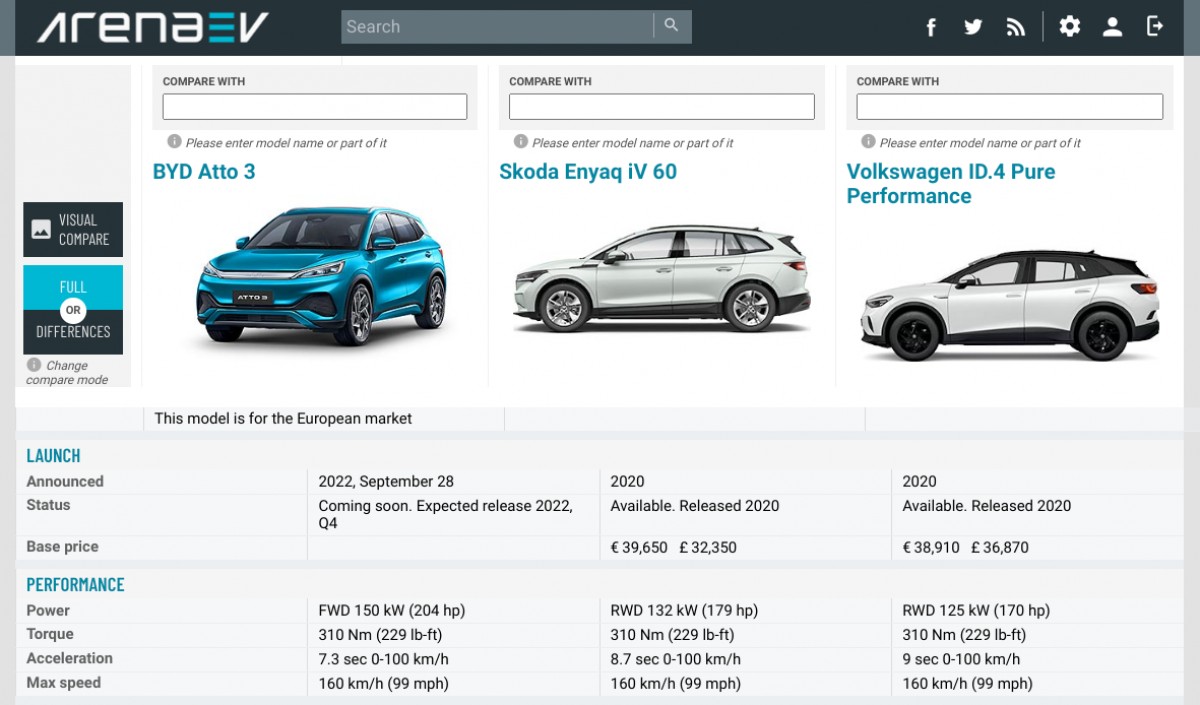This screenshot appears to be from a website or device showcasing a car comparison page. At the top, there's a black border featuring the company name "Arena EV" in white and blue text, along with a few icons for various apps and social media platforms. The white and blue text logo is modern and stylized. A gray search box centered against the black background sits in the middle of the top section. To the right, there's a row of icons including an "F" for Facebook, the Twitter bird icon, a Wi-Fi symbol, and a few other icons.

Beneath this top section, the main content of the page is divided into three centered boxes, each depicting a different car available for comparison. The cars presented are the BYD Atto 3, the Skoda Enyaq 460, and the Volkswagen ID.4 Pure Performance. Each car has its own white "Compare With" box above it. The background of the page is gray and complements the clean layout.

Each car comparison section includes a photograph of the car, followed by detailed information about its launch date and performance specifications, such as power, torque, acceleration, and maximum speed. The page appears to cut off just below these details, possibly indicating that more information might be accessible upon scrolling.